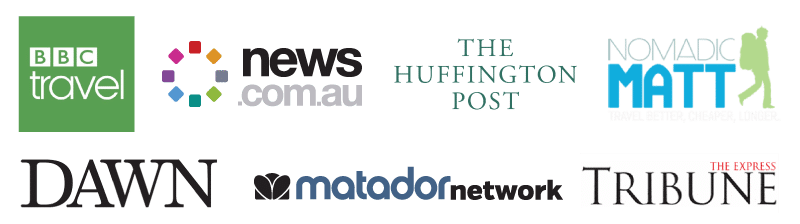This screenshot displays a collection of news site logos on a plain white background arranged in a landscape orientation across two rows of icons. 

- **First Row (Top Row):**
  1. **BBC Travel:** A green square logo located in the upper left corner.
  2. **News.com.au:** A logo with a white background featuring a small circle filled with rainbow colors next to the text.
  3. **The Huffington Post:** A simple design with a white background and the site's name.
  4. **Nomadic Matt:** Featuring teal text with "MATT" repeated twice beneath a graphic of a man backpacking towards the right.

- **Second Row (Bottom Row):**
  1. **Dawn:** The text "DAWN" in capital letters against a white background.
  2. **Matador Network:** Dark blue text on a white background spelling out "Matador Network."
  3. **Tribune:** Bold black text with "The Express" in red situated in the upper right hand corner.

Each logo represents a news site or app that the person is following, with the overall layout providing easy identification of these platforms.